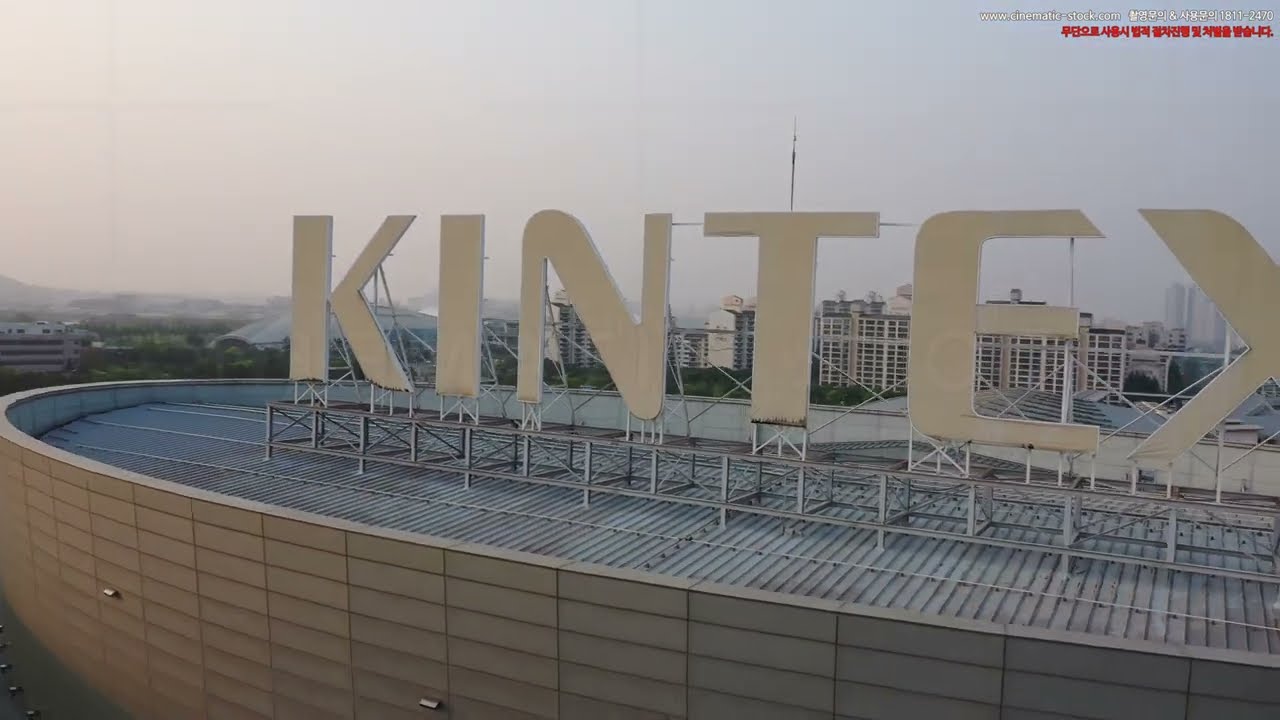The image showcases the large white, cutout letters "K-I-N-T-E-X" mounted on top of an oblong, oval-shaped building, which has a gray roof and appears to have a metal scaffold structure supporting the letters. The building resembles a stadium but is closed off. The background features several more urban buildings, including white multi-story commercial or residential structures and taller skyscrapers off in the distance. One of the buildings has a noticeable large antenna on top. The sky above is gray and hazy, with a mix of trees and hills on the left side adding to the setting. In the upper right corner of the image, there is a blurry section of text in white and red, potentially including a web address and some Asian characters, likely indicating a watermark.